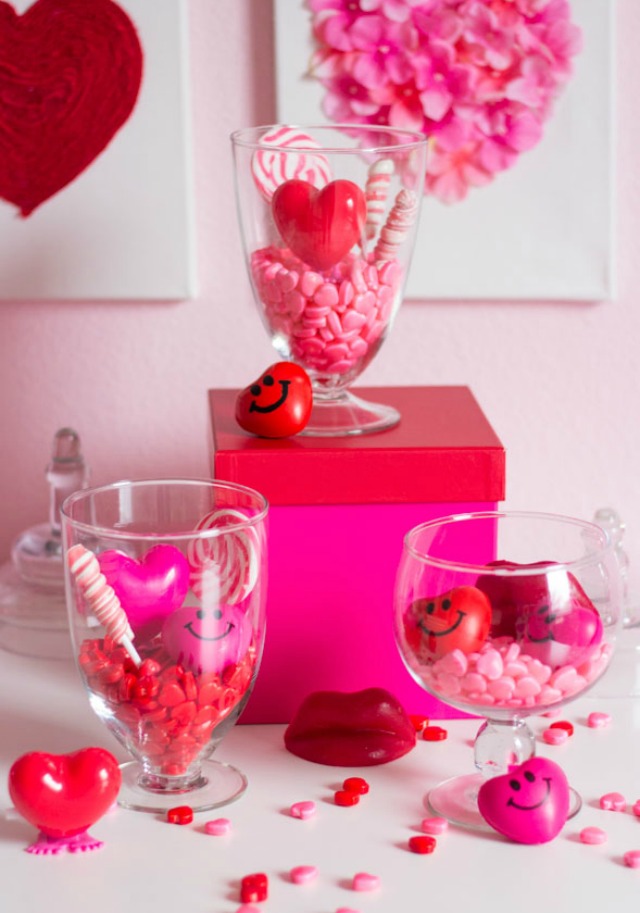The image showcases an array of Valentine's Day decorations meticulously arranged around three glass candy dishes. The background features a soft pink wall adorned with two canvases: one displays a bold red heart, while the other is a creatively arranged heart-shaped floral design. In the foreground, heart-shaped candies fill each of the glass dishes. The elevated dish, resting atop a pink and red gift box, contains red and pink heart candies, with a smiley-faced heart leaning against it. The candy dish to its left on the bottom holds red heart candies, and the dish to the right, distinguished by its shorter, unique shape, also contains pink hearts. Adding to the festive scene, red wax lips are positioned between the two lower dishes, and scattered throughout are smaller heart candies and twirly lollipops, enhancing the celebratory atmosphere. Visible on the left side of the box is a glass lid, possibly from a jar, contributing to the ensemble of whimsical, romantic décor.